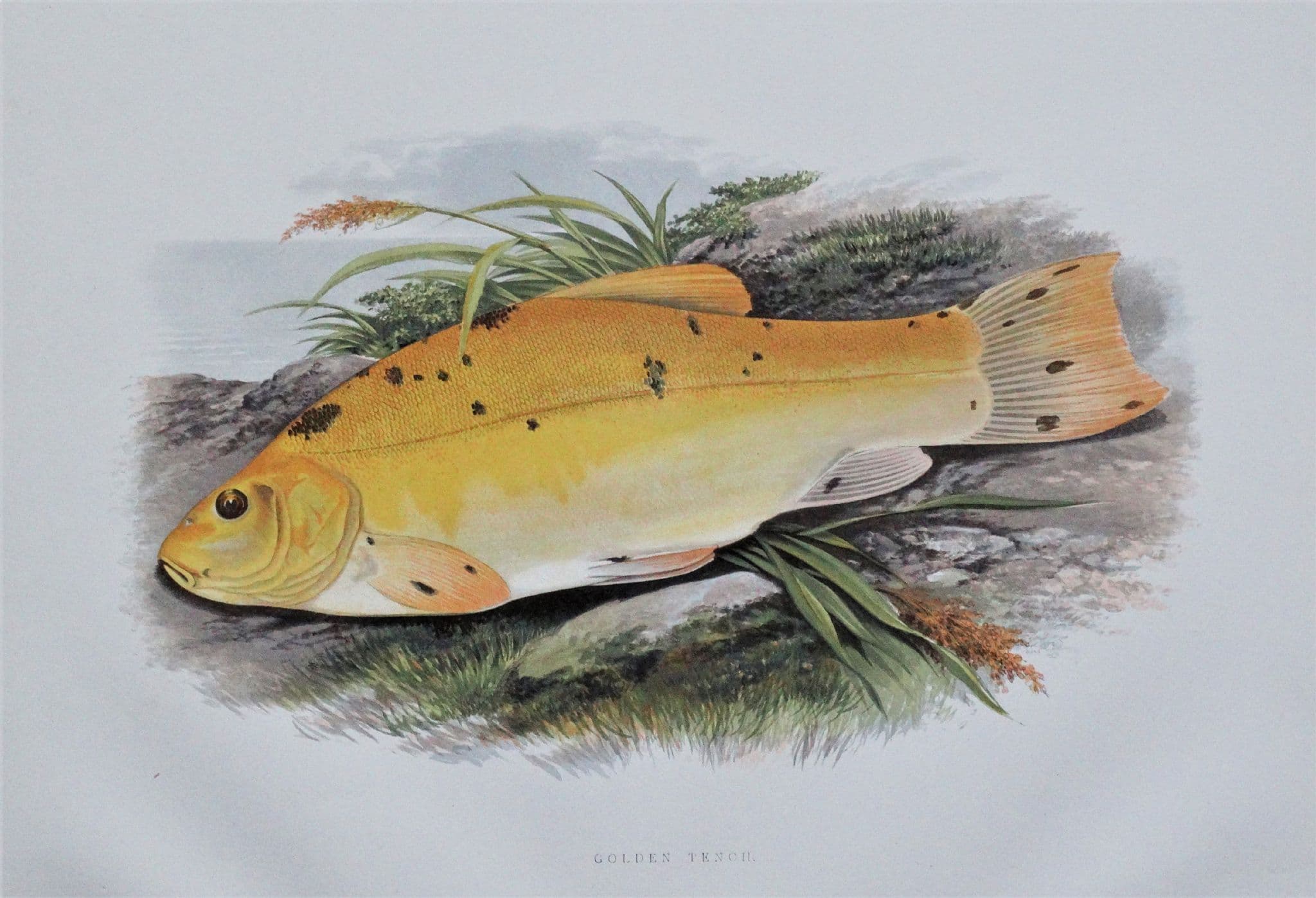This image presents a fully rendered, colored pencil drawing with a vignette effect that focuses on a central fish. The fish, which might be a "golden perch," exhibits a striking yellow-orange hue with a white underbelly and black speckles peppering its fins and tail. It lies motionless on a ground composed of grass, dirt, rocks, and plant stalks. The fish's size suggests it's meant for consumption, resembling a sunfish and measuring approximately six to eight inches. In the background, a subtle depiction of the water body and distant clouds enhances the scene, emphasizing the fish's dramatic, suspended placement amidst the natural bank. A faint text beneath the image seems to label the fish variety, though the second word is ambiguous.